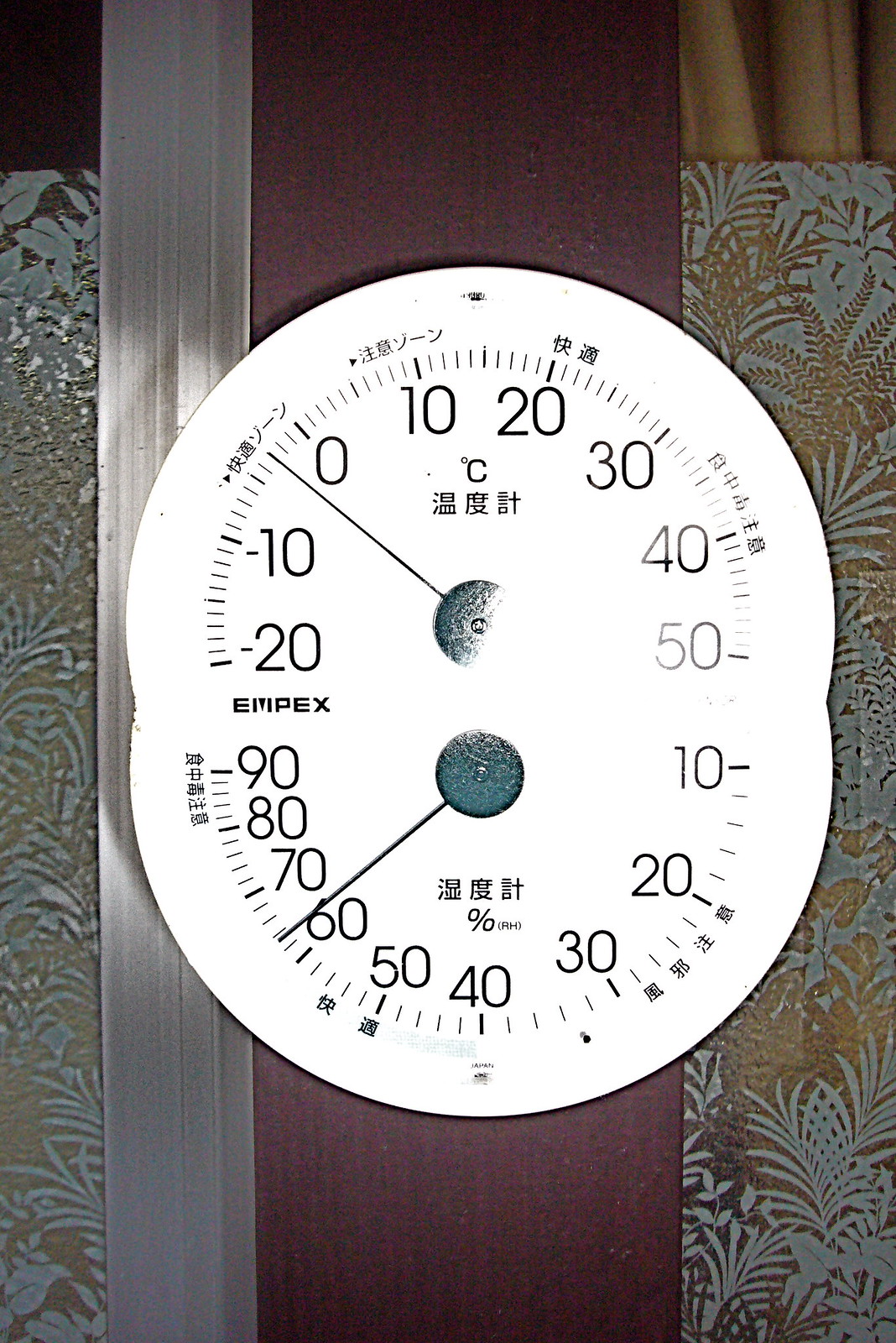This image captures a detailed view of a dual measurement instrument, likely a barometer combined with a thermometer. The top half of the device displays a circular temperature gauge marked in degrees Celsius. The temperature scale starts from -20°C on the left, rising incrementally through -10°C, 0°C, 10°C, 20°C, 30°C, 40°C, and finally 50°C. The needle appears to be pointing to approximately -3°C, indicating sub-zero temperature, which suggests the photograph may have been taken outdoors in a cold environment. The brand or model name "MPEX" is visible near the top of the scale.

Below the temperature gauge, there is another semi-circular scale that seems to measure humidity, as indicated by the word "percentage." The humidity scale starts at 10% on the far right, increasing through increments of 10% up to 90% on the far left. The needle on this gauge points to around 63%, suggesting moderately high humidity. Both scales are set within a sleek housing, and their arc shapes provide a clear and intuitive way to read the measurements.